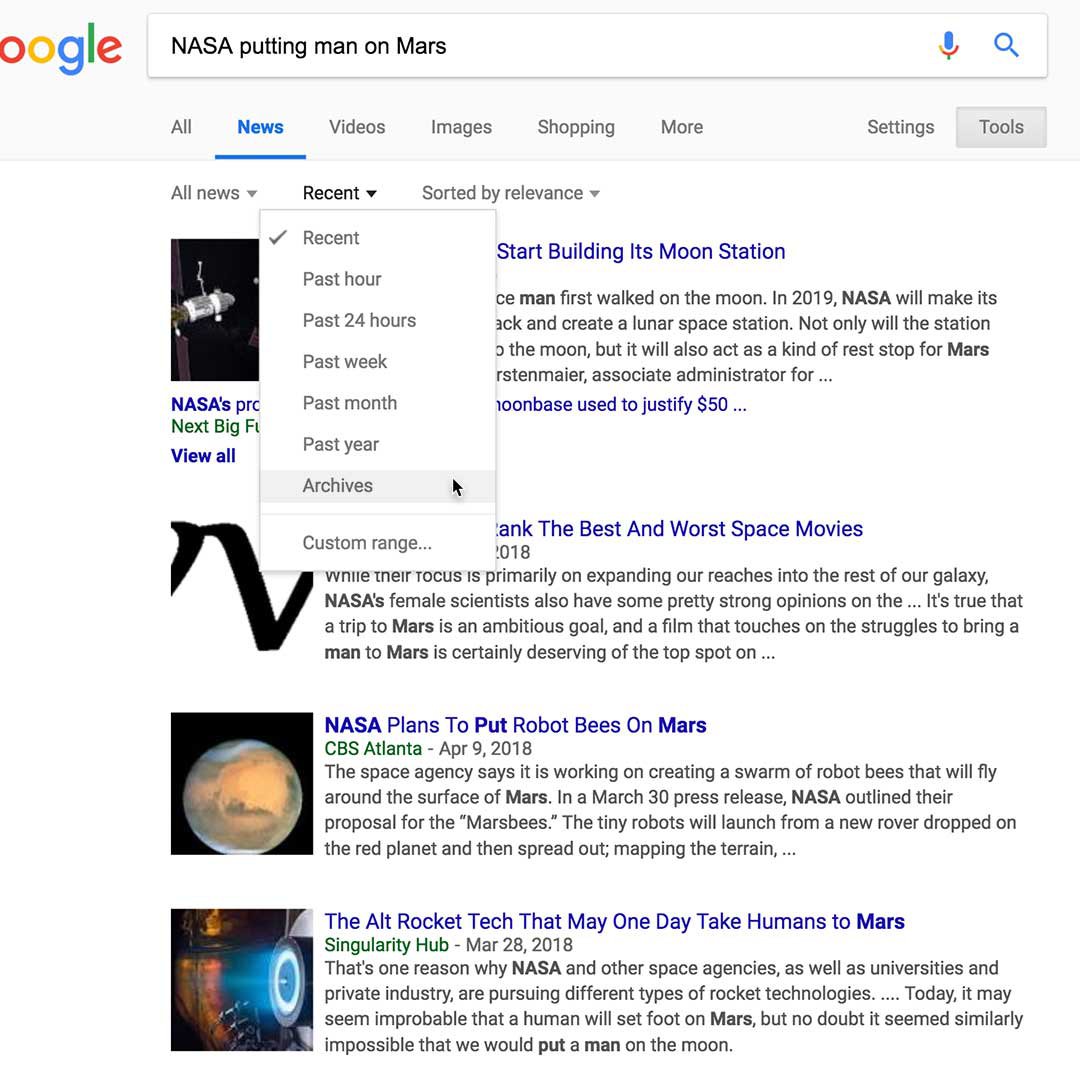The image depicts a Google search results page with the query "NASA putting man on Mars" typed into the search bar at the top. Under the search bar, various categories for refining the search results are displayed, including options such as 'All', 'News', 'Videos', 'Images', 'Shopping', and 'More'. The focus is on the 'News' category, with a drop-down menu open under 'Tools', revealing various time-related filters: 'Recent', 'Past hour', 'Past 24 hours', 'Past week', 'Past month', 'Past year', 'Archives', and a customizable date range.

On the left side of the page, there are four vertically aligned thumbnail images with brief descriptions:
1. The first image relates to the topic of NASA starting to build its moon station.
2. The second image is about the best and worst space movies.
3. The third image is a photograph of a planet, accompanied by the headline "NASA plans to put robot bees on Mars," sourced from CBS Atlanta.
4. The fourth image shows a round object emitting beams of blue light, titled "The alt rocket tech that may one day take humans to Mars," provided by Singularity Hub.

The layout is typical for a Google search results page, providing users with a range of options and visually engaging content related to the search query.